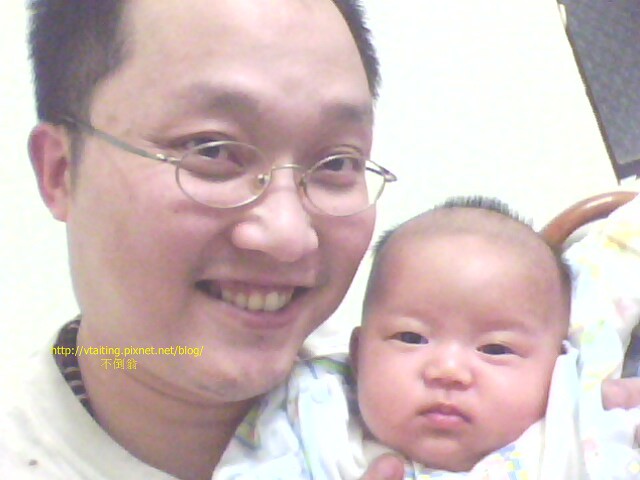This close-up photograph captures a joyful moment between an Asian man and a baby, likely his own. The man, who has short dark hair and a very high hairline, is wearing oval glasses and is smiling broadly, displaying a big, toothy grin. He is partially dressed in what looks like a white t-shirt with another shirt underneath. The baby, also appearing to be of Asian descent, is wrapped snugly in a swaddling blanket that is primarily white with yellow design patterns. The baby, who has little patches of hair popping up on its head and big, puffy cheeks, looks to be a few months old rather than a newborn. Both their heads fill most of the image, with the baby's face positioned to the right of the man (to the viewer's left). The background is mostly indistinguishable due to bright lighting, though there are hints of a white wall and possibly some dark curtains or a dark object to the right. The top of the image features text that reads "http://phytylene.pixnet.net/blog."